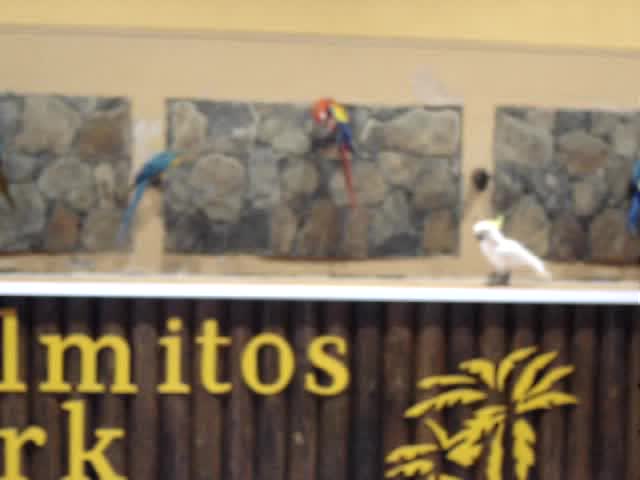The photograph depicts a trio of birds in what appears to be a zoo or exhibition setting, characterized by its artificial, decorative environment. The central bird is a vibrant parrot with a plumage of blue, red, and yellow, perched on a middle perch. To the left of the parrot is an all-blue bird with a long tail, also perched but on a slightly lower wooden stick. The third bird, a white cockatoo distinguished by a prominent yellow feather atop its head, is positioned on the ground. The background features three panels of a faux rock wall. Below the birds runs a white shelf-like platform, beneath which there is a distinctive bamboo wall. On this wall, partially visible yellow letters spell out "CLMITOS" followed by "RK." To the right of this signage, there is a decorative element resembling a palm tree or palm leaves made from the same material as the letters.